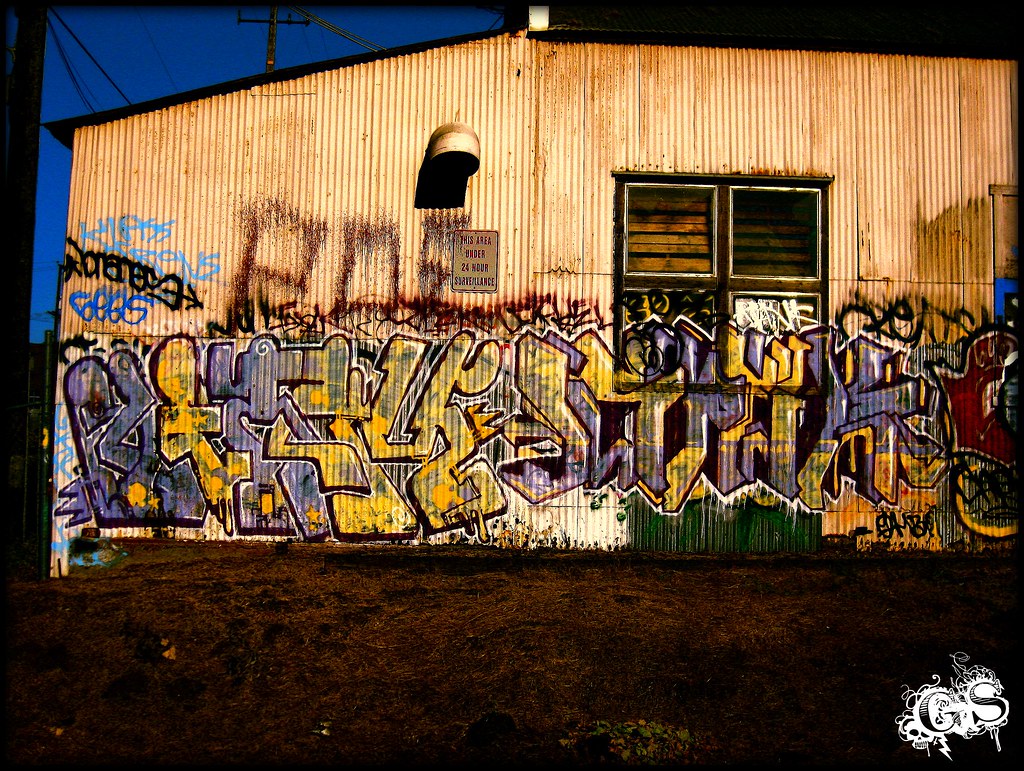The image depicts the side of an old, potentially abandoned warehouse constructed from corrugated metal with a tan, often rust-stained exterior. The photograph is taken from a ground perspective looking slightly upward, capturing a portion of the dark blue evening sky above. The building features a slanted roof on the left side and a window with four glass panes and a dark brown or white frame off-center to the right. The lower half of the wall is extensively covered in graffiti, primarily in purples and yellows, consisting of abstract figures, pseudo letters, and some lines and scribbles in red, blue, and black that blend together. At the bottom right corner of the graffiti, there is a noticeable watermark that features the capital letters "G.S." on a white background. The base of the building rests on dark brown dirt, with a foreground scattered with dried grasses or hay.